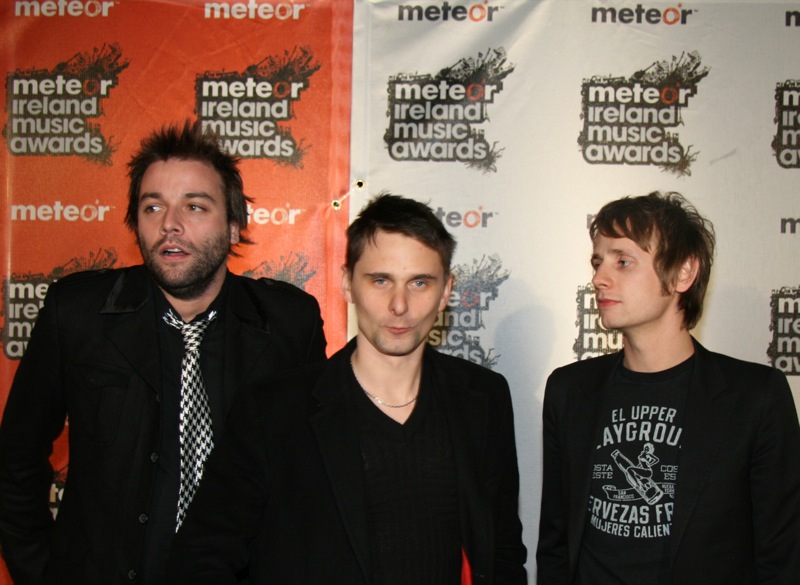In the image, three men are prominently standing against a backdrop for the Meteor Ireland Music Awards, which features a repeated logo that alternates between an orange background on the left and a white background on the right. 

The man on the left stands out with his spiky dark hair and wears a black outfit accentuated by a houndstooth-patterned black-and-white tie. He is looking to the left and has a beard and mustache. 

The man in the center is dressed entirely in black, complemented by a gold necklace. His short brown hair frames a face where he's sucking in his cheeks. 

On the right, the third man sports a black jacket over a black t-shirt adorned with white text and an image. His mid-neck-length brown hair faces the man in the middle, creating a slight interaction between them. 

None of the men are smiling as they pose for this awards event photo.